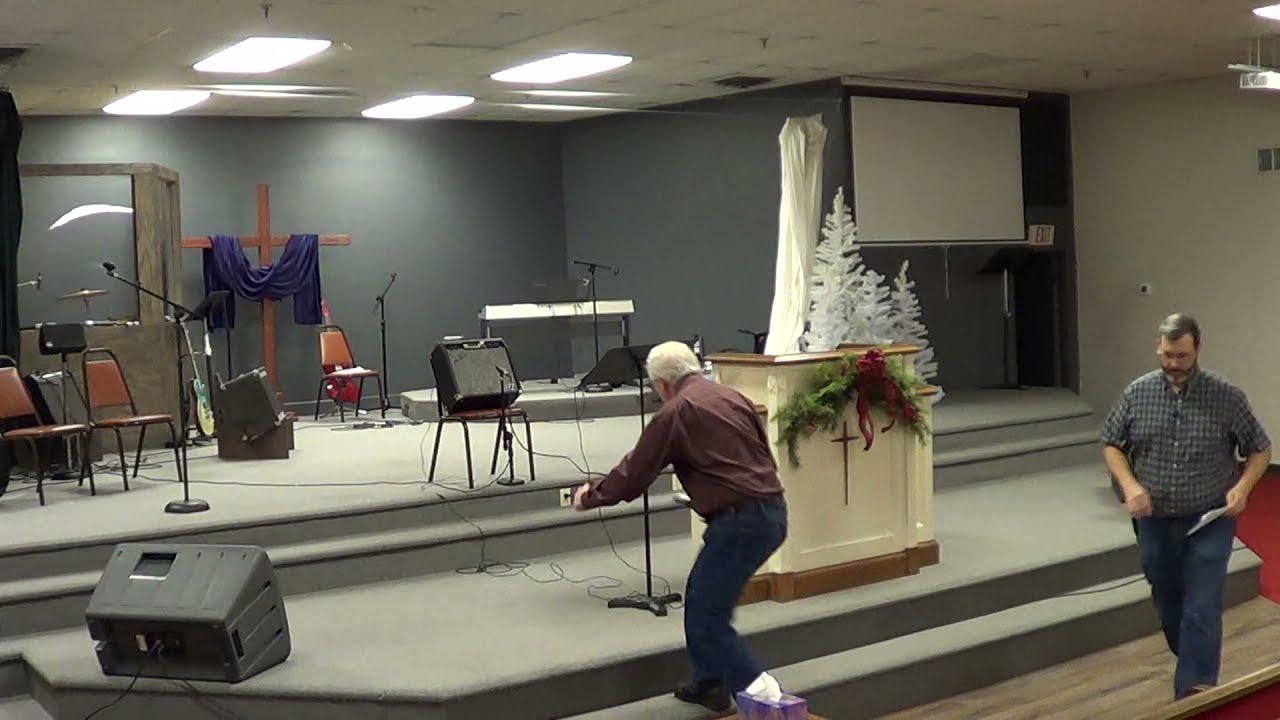The image captures the interior of a church, focusing on the platform area, which appears to be undergoing some preparation before a service. The scene is detailed with white-paneled ceilings and four fluorescent lights positioned at the back of the stage. The back wall of the stage is painted gray, contrasting with the tan walls off the stage. At the center back of the platform, a brown wooden cross adorned with a purple scarf rests on the floor. 

The platform itself is divided into two levels, accessed by two sets of steps. On the lower level, a large wooden podium featuring a Christian cross and wreath stands prominently. Surrounding the podium, there is a mix of musical equipment, including speakers, microphone cords, a keyboard piano, a portion of a drum set, and a guitar. Three brown chairs with black frames and various speakers are arranged on the upper stage. 

In the foreground, one man with silver hair, dressed in a long-sleeved purple shirt and jeans, is bent over, adjusting some microphone cords. Another man, wearing a plaid shirt and blue jeans, is walking behind him, possibly heading towards the stage area. The image is brightly colored and devoid of additional people, emphasizing the peaceful, preparatory moment inside the church.